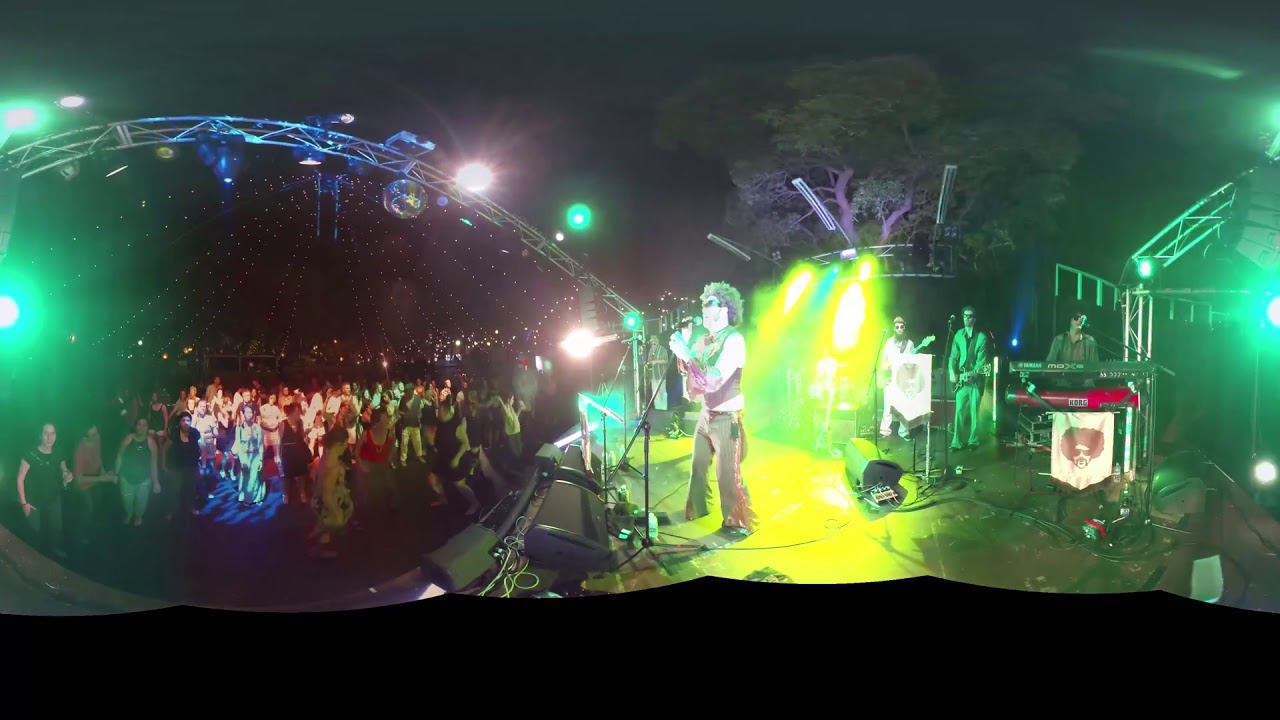This vivid nighttime photograph captures the electric atmosphere of a live rock concert, showcased through a 360-degree panoramic view. The image expertly stitches together multiple shots, providing a comprehensive portrait of both the energetic stage and the enthusiastic crowd. 

On the right-hand side, the stage is bathed in green and yellow spotlights that illuminate a dynamic scene. At the forefront, a man with dark, fluffy hair sings passionately into a microphone mounted on a stand, his face overexposed to a glowing white due to the intensity of the lights. He grips the mic with both hands, pouring his energy into his performance. 

Behind him and slightly to the side, the stage features a bass player and two guitarists. The guitarist closest to the audience sports a gray suit and a black shirt, while the keyboard player, dressed in a brown button-down shirt, commands two keyboards positioned in front of him. Each musician has a microphone nearby, suggesting they contribute vocally as well.

An imposing metal arch with numerous lights is poised in front of the stage, though these lights are currently off, hinting at a thrilling potential for a sequenced light show later in the concert. Floor monitors are strategically placed to ensure the performers can hear themselves clearly.

Shifting focus to the audience on the left side of the image, a bubble-like effect creates a distinctive visual where spectators appear to shift in size and distance, adding to the panoramic drama. The crowd, predominantly female and standing, dance and sway beneath the varied lighting. Overhead, the stage lights are mounted on a domed structure that weaves in and out of sight due to the image stitching, imparting a wave-like effect.

The stitched-together photo even highlights a large tree behind the stage, encircled by a metal structure adorned with unlit lights, adding a natural yet structured element to the concert setting. This detailed portrayal captures the vibrant essence of the event, from the performers' intense focus to the audience's unbridled joy.